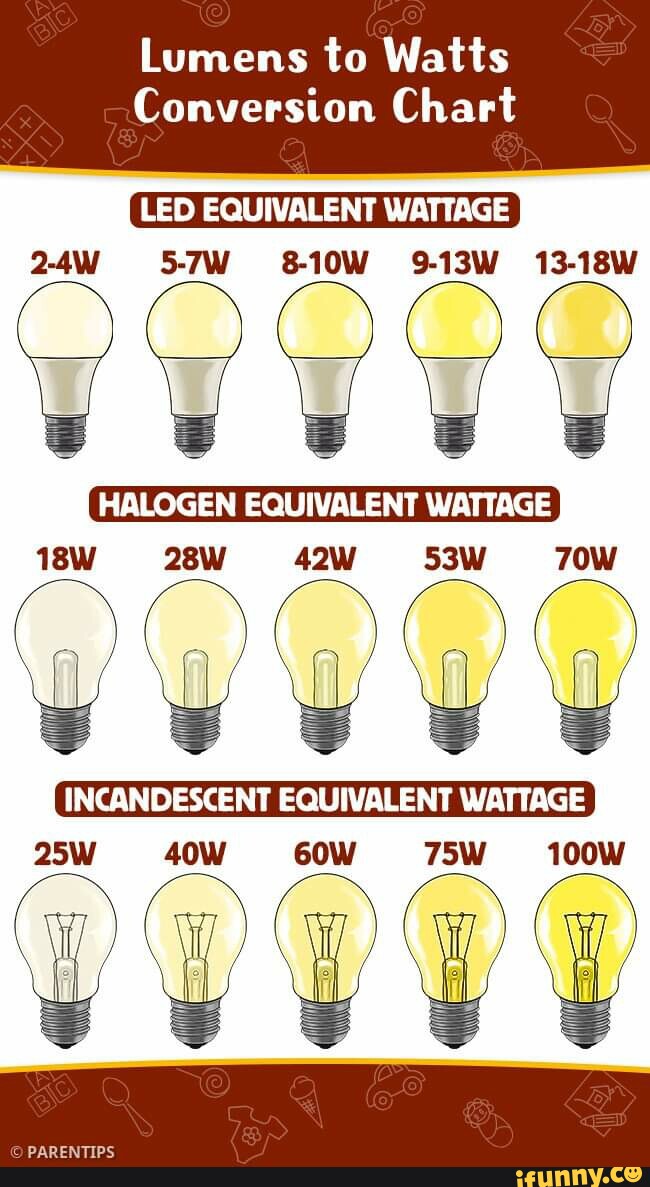This image is a detailed Lumens to Watts Conversion Chart, prominently titled in brown at the top. The chart features three rows of light bulbs, each representing different types of equivalent wattages. 

The first row is labeled "LED Equivalent Wattage" and showcases five light bulbs with wattages ranging from 2-4 watts, 5-7 watts, 8-10 watts, 9-13 watts, to 13-18 watts. Each bulb emits light in shades of yellow, deepening with higher wattages.

The second row lists "Halogen Equivalent Wattage," also with five light bulbs. The halogen bulbs have wattages of 18 watts, 28 watts, 42 watts, 53 watts, and 70 watts, transitioning from a pale whitish-yellow to a bright yellow as the wattage increases.

The third row is titled "Incandescent Equivalent Wattage" and includes five light bulbs ranging from 25 watts, 40 watts, 60 watts, 75 watts, to 100 watts, with the color of the light deepening to a bright yellow at the highest wattage.

At the bottom of the chart, it is copyrighted by "Parent Tips" and mentions "ifunny.com". This visual guide effectively cross-references the power equivalents among LED, halogen, and incandescent light bulbs.